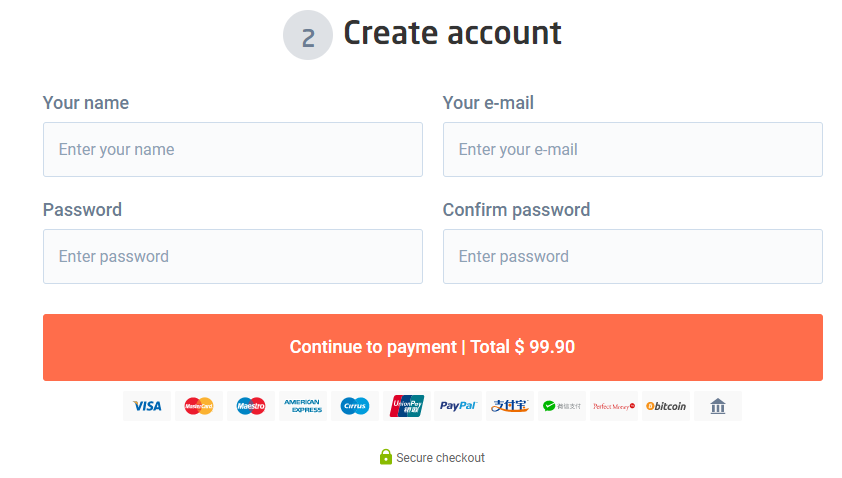The image depicts a user interface for creating an account and proceeding to payment.

At the top, there's a gray circle with a gradient transitioning from blue to gray. Next to it, the text "Create Account" is displayed. Below, there are several input fields for user information:
- A text box labeled "This is your name" with a placeholder text "Enter your name."
- A text box labeled "Your email" with a placeholder text "Enter your email."
- Two text boxes for password entry: "Password" and "Confirm Password," each with the placeholder text "Enter password."

Below these fields, an orange button with white text reads "Continue to Payment - Total: $99.90."

Under the button, a comprehensive list of payment options is displayed:
- Visa
- MasterCard
- American Express
- Citibank
- PayPal
- An unfamiliar Chinese payment option with blue Chinese characters and a yellow swish
- Bitcoin
- A symbol resembling a gray building, likely representing bank transfer

At the bottom of the image, a green padlock icon signifies a secure checkout. The background of the entire interface is white.